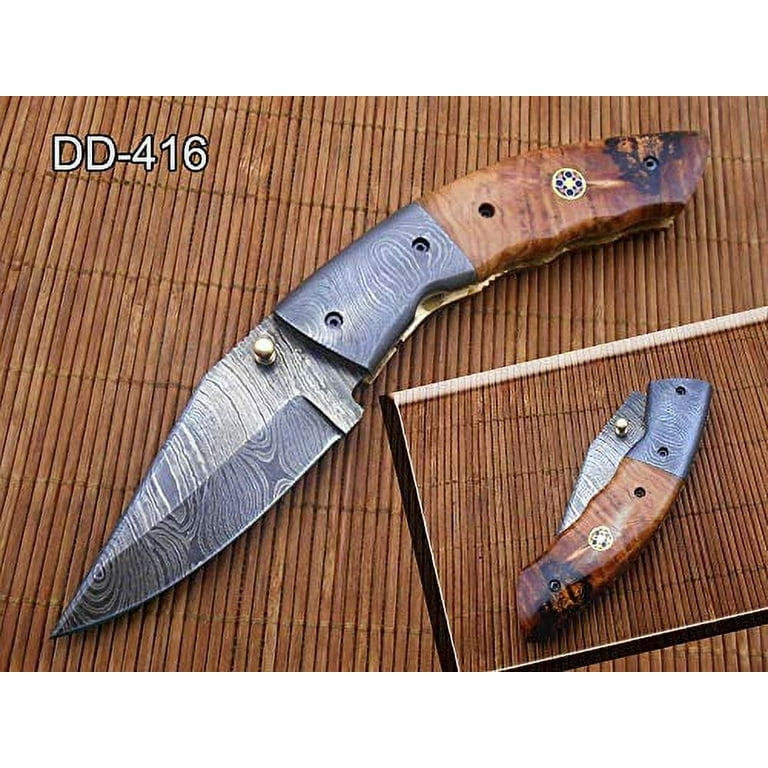A detailed image showcases a high-quality knife in two different orientations. The backdrop for the photograph is a rustic, brown wooden mat, enhancing the knife's craftsmanship. In the upper left corner of the image, the designation "DD-416" is elegantly inscribed in white font. 

The centerpiece of the image features the knife in its open configuration. The knife boasts a sturdy brown handle, seamlessly integrated with a sleek silver bolster, leading to a sharp, polished silver blade. 

In the lower right corner, a smaller inset image presents the knife in its folded state, with the blade securely tucked inside the handle, highlighting its practical, portable design. This composition effectively showcases both the aesthetic appeal and functionality of the knife.